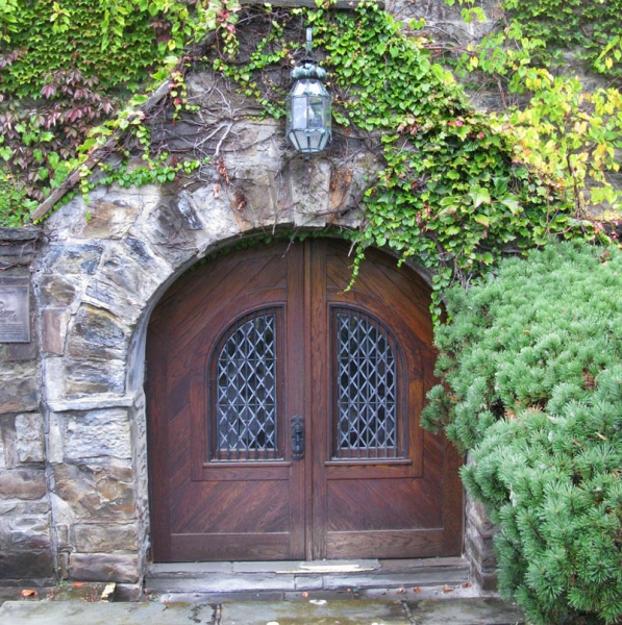The image showcases an enchanting, Hobbit-like scene with a small, arched, brown wooden door set into a gray, brown, and white stone building. The door, evocative of something straight out of Lord of the Rings or The Hobbit, features decorative windows with crisscross designs that add to its charming, old-world character. The building's facade is blanketed in lush greenery, with moss and leaves climbing the stone walls and a cluster of green bushes framing the right side of the door. Above the door, a glass light fixture hangs, poised to illuminate the entrance at night. The ground in front of the door is partially visible, revealing a bit of concrete. The primary colors in the image are the earthy browns of the door and stones, intertwined with the vibrant greens of the foliage, creating a picturesque and serene atmosphere.